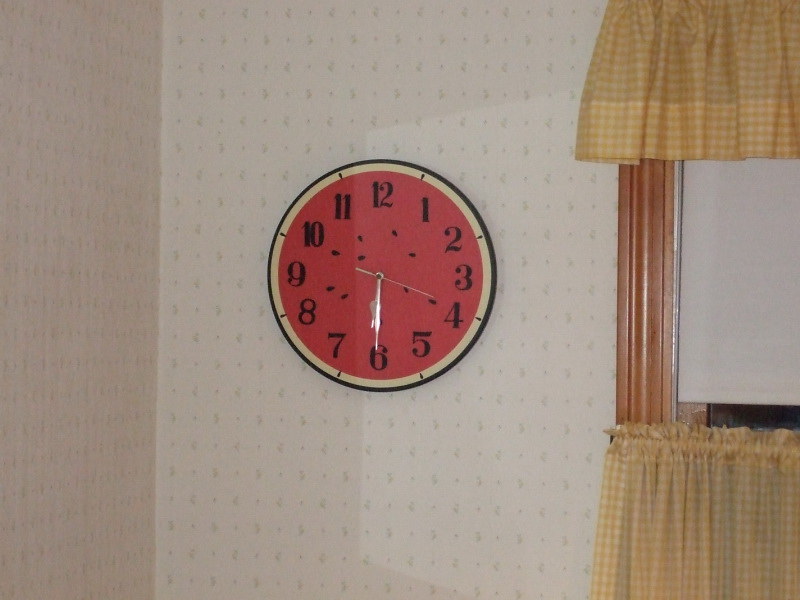The photograph features a charming, contemporary-styled wall clock designed to resemble a slice of watermelon. The clock, positioned near the center of the image, showcases a thin green outer ring followed by a thicker white ring, and a vibrant red face speckled with black dots mimicking watermelon seeds. The numerals are traditional, black, and encircle the face, with silver hour, minute, and second hands pointing respectively to the 6 and the 4. The room has a retro aesthetic, accentuated by the wallpaper which is white or cream with an indistinct green pattern. To the left of the clock is a window framed in wood, adorned with yellow and white checkerboard cafe curtains at the top and bottom, alongside a partially pulled-down white blind. The photograph, likely taken with the help of interior lighting, captures the quirky yet endearing details of this whimsical wall clock within the cozy setting.